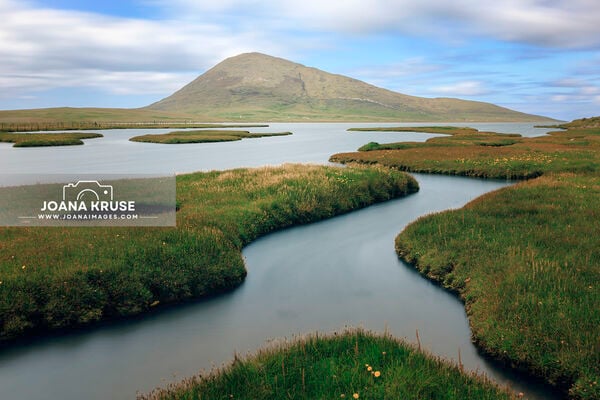This captivating nature photograph, taken by Joanna Cruz (www.joannaimages.com), showcases a stunning outdoor landscape brimming with vibrant details. In the background, a majestic, green and gray mountain stands tall against a brilliant blue sky dotted with white clouds. The foreground teems with an intricate network of waterways and winding creeks, punctuated by soft patches of tall, bright green grass interspersed with colorful flowers in shades of yellow, pink, and orange. These waterways begin about one-third down from the top of the photo and snake their way through the raised areas, creating little round islands of lush vegetation. On the left side of the image, a transparent gray rectangle features an iconic camera graphic along with the photographer's name, Joanna Cruz, and her website, www.joannaimages.com.